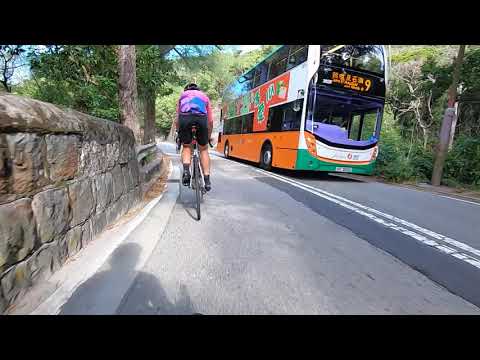The image depicts a vibrant outdoor scene of a road viewed from a bike lane. On the left side, a cyclist, wearing a pink and blue jersey and black shorts, is pedaling up a hill with both hands on the handlebars. Adjacent to him, a stone wall and a railing border the lane, lined with various trees and a small strip of blue sky visible at the top. On the opposite side of the road, a large double-decker commuter bus with black windows, orange and green sides, and an electronic sign displaying the number 9 travels downhill towards the viewer. The bus also features Asian lettering on a red billboard. A light pole is situated on the right side of the road, which also has some shrubbery. Shadows cast by the cyclist suggest the presence of additional people, adding to the dynamic nature of this rural setting.